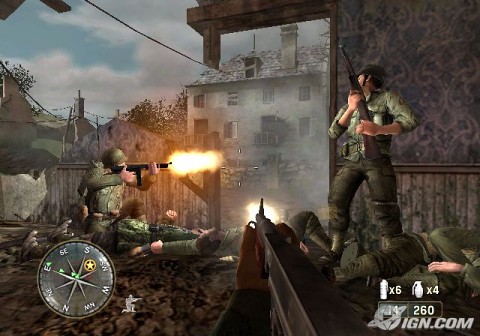A highly detailed and ultra-realistic image captured from a video game depicts a chaotic war scenario. Amidst the rubble of a city ravaged by battle, two soldiers are entrenched in the heat of combat. The desolate urban landscape features the remnants of buildings, their windows shattered and facades stained with smoke and fire damage. One soldier, clad in full army uniform and helmet, is crouched in a squatted position, firing an automatic rifle, with a vivid muzzle flash visible. Nearby, another soldier takes cover behind a crumbling wall, gripping his rifle upright and ready. The intensity of the scene is underscored by a compass displayed at the bottom of the screen, adding to the immersive experience. The detailed destruction and precise depiction of the soldiers reflect the game's advanced graphics and intense atmosphere.